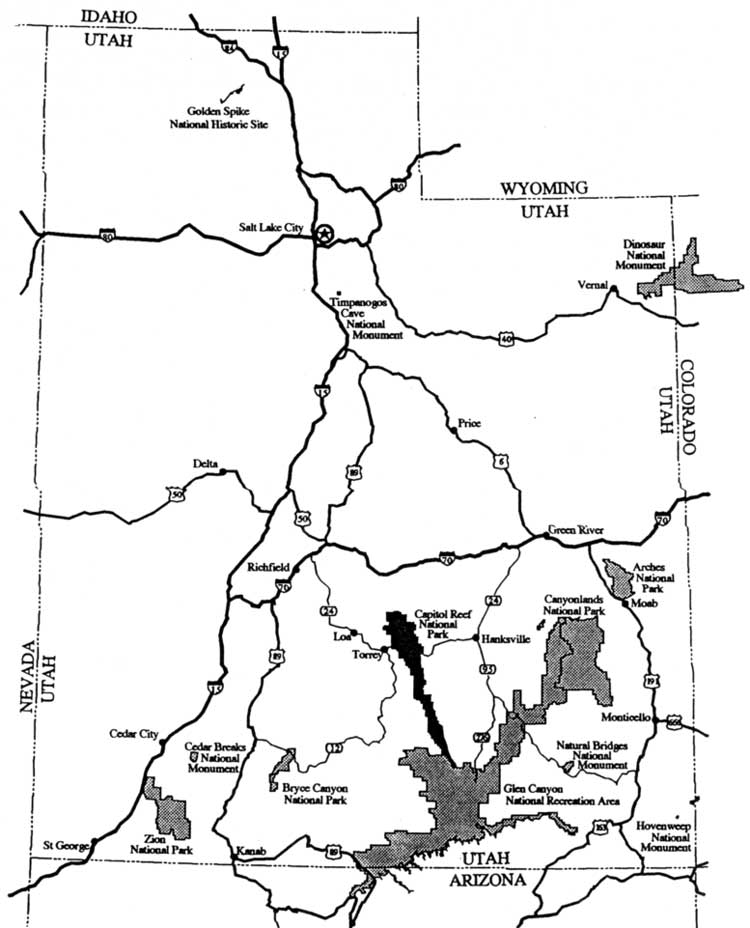This detailed black and white map focuses on the state of Utah, displaying its borders with Idaho to the north, Nevada to the west, Arizona to the south, and Colorado to the east, with Wyoming nestled at the northeastern edge. The borders of these neighboring states are depicted with dotted black lines. Major highways cris-cross the state, including Interstate routes that are slightly blurry but identifiable as 50, 80, 15, 84, and 6.

Salt Lake City, marked with a star near the center towards the top, stands out among various other city markers. Significant landmarks such as the Golden Spike National Historic Site appear near the top left. The map highlights several national parks, including Capitol Reef, Canyonlands, and Bryce Canyon, with shaded areas indicating their locations. The map foregoes a focus on large metropolitan areas, concentrating instead on the state's roadways and natural landmarks, delineated in clear, black text.